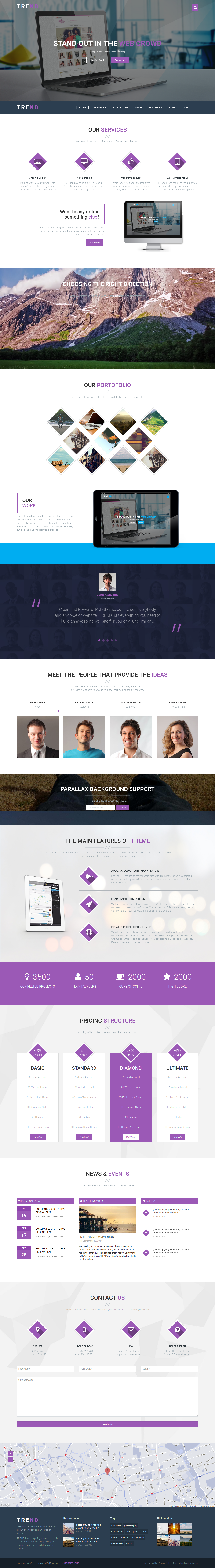This is a detailed description of a compressed website template designed for mobile viewing:

The website template designed for mobile viewing presents a compressed vertical layout that distorts the aspect ratio, causing all elements to appear squashed together. At the top, there is a hero image with a dark overlay featuring the text "Stand Out in the Crowd" with "Crowd" highlighted in purple. 

Below this are four icons set within diamond shapes under the section labeled "Our Services." This is followed by a section titled "Choosing the Right [Something]" placed over an image of snow-capped mountains with clouds and a tree-filled field at the base.

Further down, there is a grid forming an interlocked chain-link pattern, comprising four diamonds in the first row, three in the second, and four in the third. Beneath this grid, a smartphone is displayed on its side, leading into a footer that contains a quote next to a person's photo.

The next section highlights a team introduction with the header "Meet the People Who Provide the Ideas." It features photos of four individuals—three men and one woman, all Caucasian. Their attire varies: the first man is in a suit, the second in a blue t-shirt, the third in a white dress shirt without a tie, and the woman in a black dress.

Following the team section, there's a mention of "Parallax Background Support," accompanied by a screen image and various bullet-pointed icons to the right. Below these icons, various numbers such as 3,500, 52,000, and 2,000 are displayed, likely indicating statistics or installations.

The template then breaks down the pricing structure before moving to the "Contact Us" area. At the bottom, there is an inserted Google Map, followed by the footer section that likely contains tags and social media screenshots.